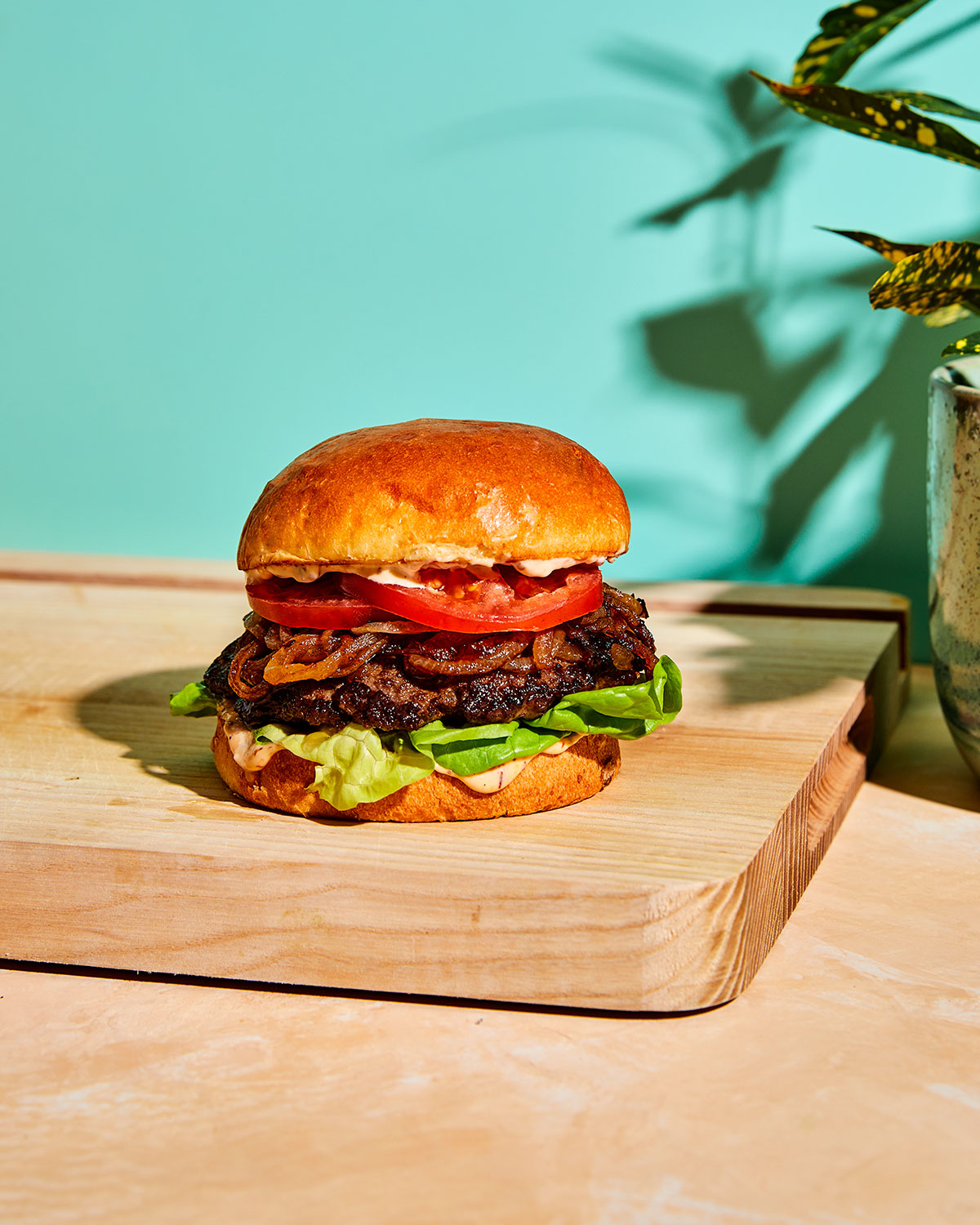This detailed photograph features a meticulously crafted hamburger set on a rectangular wooden cutting board. The base of the photograph shows a tan-beige tabletop accented with white streaks. The burger, centered on the cutting board, showcases a beautifully golden-brown top bun with hints of orange. Generous layers of sliced tomato and dark caramelized onions rest atop a charred hamburger patty. Fresh lettuce is layered beneath the patty, with a white sauce, likely mayonnaise, drizzling from beneath it. The bottom bun is a crisp gold color. The background is softly blurred, directing focus to the burger, and features a turquoise wall with a hint of green house plants peeking in from the right. The vivid colors and bright lighting give the hamburger an appetizing and professionally-styled appearance, comparable to those seen in high-end food advertisements.